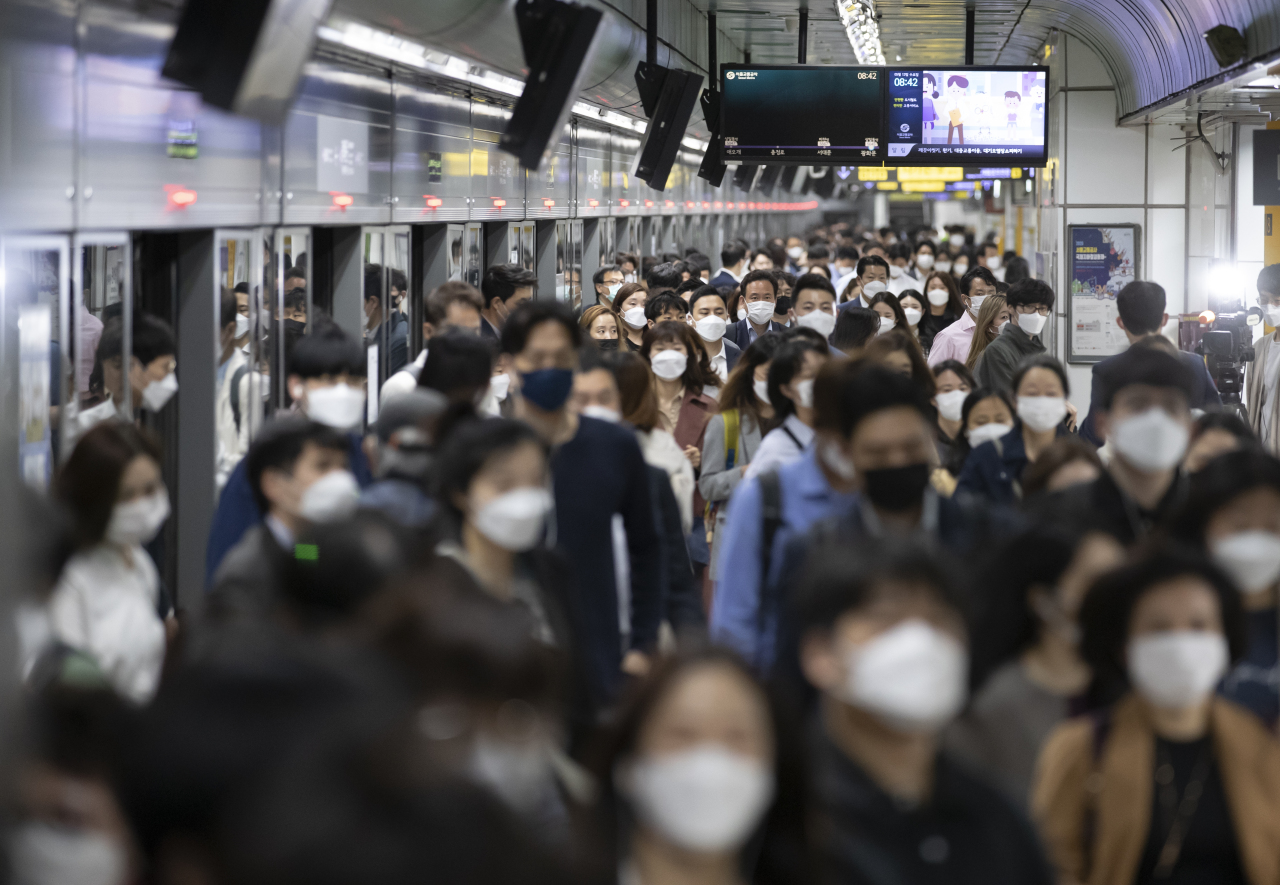The image depicts a densely packed subway car or station teeming with people, all wearing face masks, predominantly white with a few black or blue ones interspersed. The majority appear to be of Asian descent and dressed in business attire. The crowd is shoulder to shoulder, facing various directions but generally oriented towards the front of the image. To the left side of the image, red lights and subway or train doors are visible, contributing to the bustling atmosphere. Ahead, a TV screen displays a cartoon, while adjacent screens provide information on train schedules. On the top right, a curved structure with lines leads towards the ceiling. Additionally, there's a camera filming the scene, partially visible on the right side of the photo. The overall scene conveys a sense of urgency and high volume of commuters, characteristic of a busy metropolitan subway station.